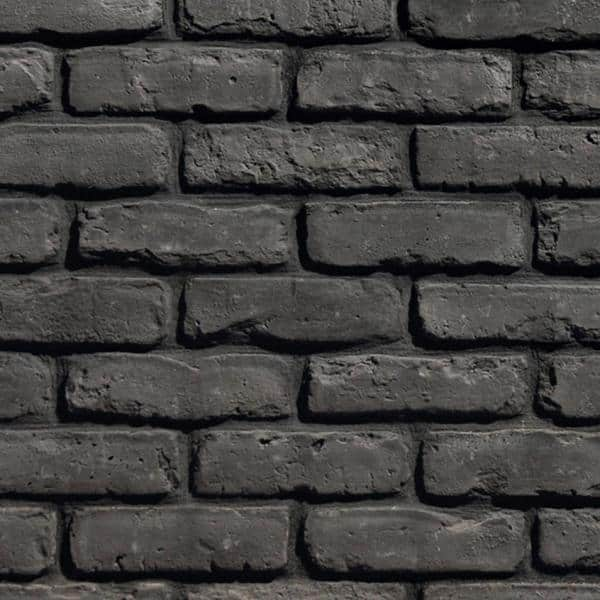The image features a section of a gray brick wall laid in a traditional, staggered pattern, where the center of one brick aligns with the joint of two bricks below it. The bricks and the mortar are both a dark gray color, suggesting that the wall might have been spray-painted. The wall is roughly three bricks wide and eight bricks tall, with each brick showing significant signs of wear and irregularities. Some bricks have chips and curved edges, deviating from the perfect rectangular shape, and exhibit a rough texture. Certain bricks appear shiny, hinting that they might have been painted over. The overall construction looks tidy despite the imperfections in individual bricks, with the specific wall surface not revealing what structure it belongs to.